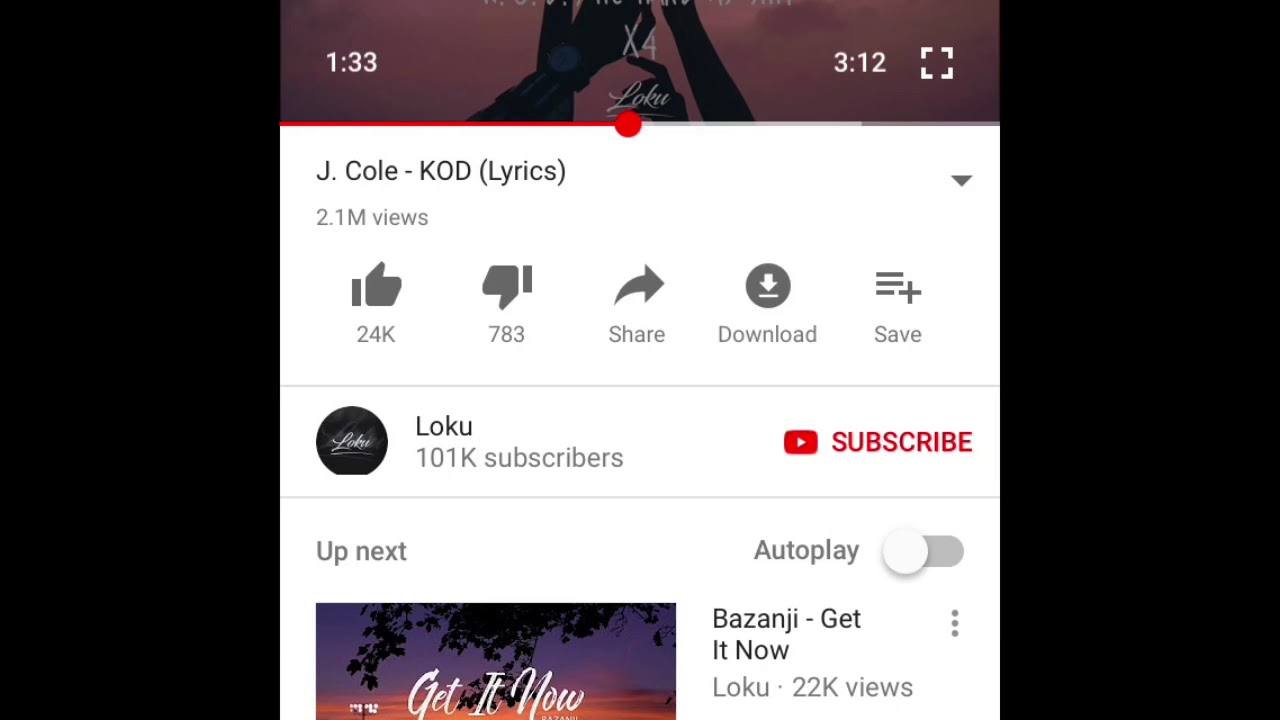The image is a screenshot displaying YouTube video information. This screenshot has black pillar boxes on both the left and right sides, framing the central content. At the top fifth of the screen, there's a pinkish-purple, cloudy background, featuring a silhouette at the bottom. Faded white text overlaying this background reads "X4 Loku."

Below this is a progress bar that is about halfway filled. The left half of the bar is red, transitioning to white, and then gray towards the far right. A red dot marks the current position on the progress bar, situated at the center.

Overlaying the video on the left side is white text displaying "133," and on the right, it shows "312." To the right of this text is a full-screen icon.

Directly below the video is a white background providing more detailed information. At the top, it indicates the video title: "J. Cole, KOD (K-O-D, all caps) Lyrics." Underneath, the view count is specified as "2.1 million views." Following this, a thumbs-up icon denotes 24K likes and a thumbs-down icon displays 783 dislikes. Next to these, icons for sharing, downloading, and saving are placed. The share icon is an arrow pointing to the right, the download icon is a gray circle with a white arrow pointing down at a horizontal white line, and the save icon shows three rows of gray lines with a plus button.

Further down, the publisher name "Loku" is displayed along with a black circle featuring "Loku" in white cursive text. The channel has "101K subscribers" noted to the right of this, alongside a red subscribe button.